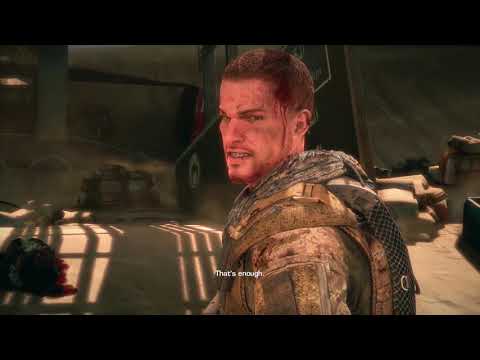This is a highly detailed screenshot from a realistic war-themed video game, presented in full color and in a horizontally rectangular frame with black borders on the top and bottom. The focus is on a wounded, white male soldier with a short brown buzz cut and a trimmed beard. His face, marked by blood, dirt, and an injury to his left temple, shows a grimace with gritted teeth, revealing a sense of anger or defiance. He is viewed from his side but is tilting his head to look directly at the viewer with slightly open eyes and mouth. 

The soldier is dressed in a thick military suit, possibly made of leather or a similar durable material, and around his neck, scarves flow from the back of his hood. He seems to carry a backpack or a parachute pack. The backdrop displays a dusty, desert-like environment with visible sandbags or containers and some shadowed structures, contributing to the war-torn ambiance. 

The image features white text at the bottom, akin to subtitles, stating, "that's enough." This suggests either the character's dialogue or a narrative cue, emphasizing the tension of the scene.